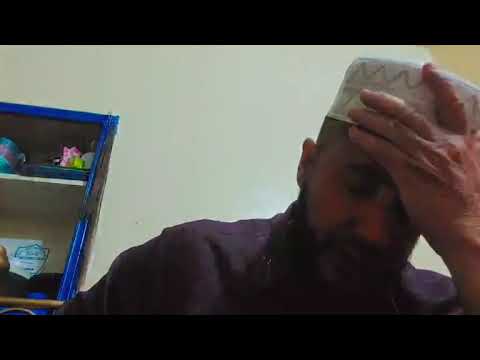The image depicts a man of Middle Eastern descent, possibly Muslim, sitting indoors against an off-white wall and a blue bookshelf. The man is positioned on the right side of the horizontal photograph, which is letterboxed with black bars at the top and bottom. He is wearing a white round cap or turban and a long-sleeved purple shirt. He appears to be very distressed or deep in thought, with his eyes closed and his left hand resting on his forehead, partially covering his face. His expression suggests frustration or sadness. The background features a blue bookshelf on the left side of the image, holding several of the man's possessions including a light blue and pink cup, a pink object, and a clear glass shield or award with a blue design. The overall tone of the image is quite dark, adding to the somber mood.